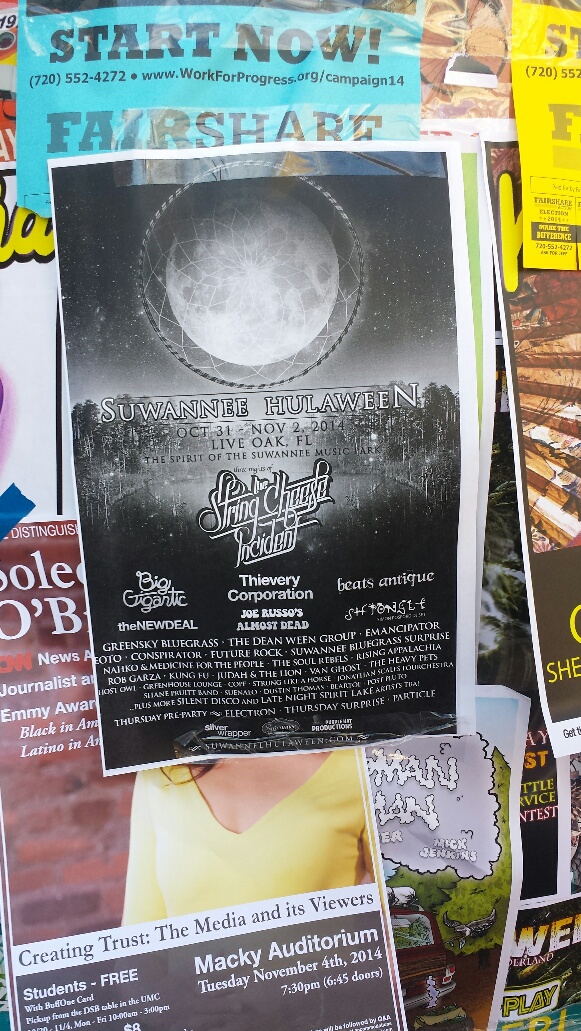The image features a wall plastered with numerous event flyers, with the central flyer prominently advertising the Suwannee Hulaween festival. This main flyer, set against a dark background, depicts a moon encircled by a dreamcatcher-like wreath, framed by stars, with a ghostly silhouette of houses among trees in the background. White text across the flyer announces "Suwannee Hulaween" with dates from October 31st to November 2nd, 2014, at Live Oak, Florida's Spirit of the Suwannee Music Park. Headliners for the event include The String Cheese Incident, Thievery Corporation, The New Deal, Big Gigantic, Beats Antique, and Joe Russo's Almost Dead. Beneath and around this main flyer, additional posters and advertisements for various other events and services are visible, contributing to the vibrant, cluttered aesthetic of the wall.